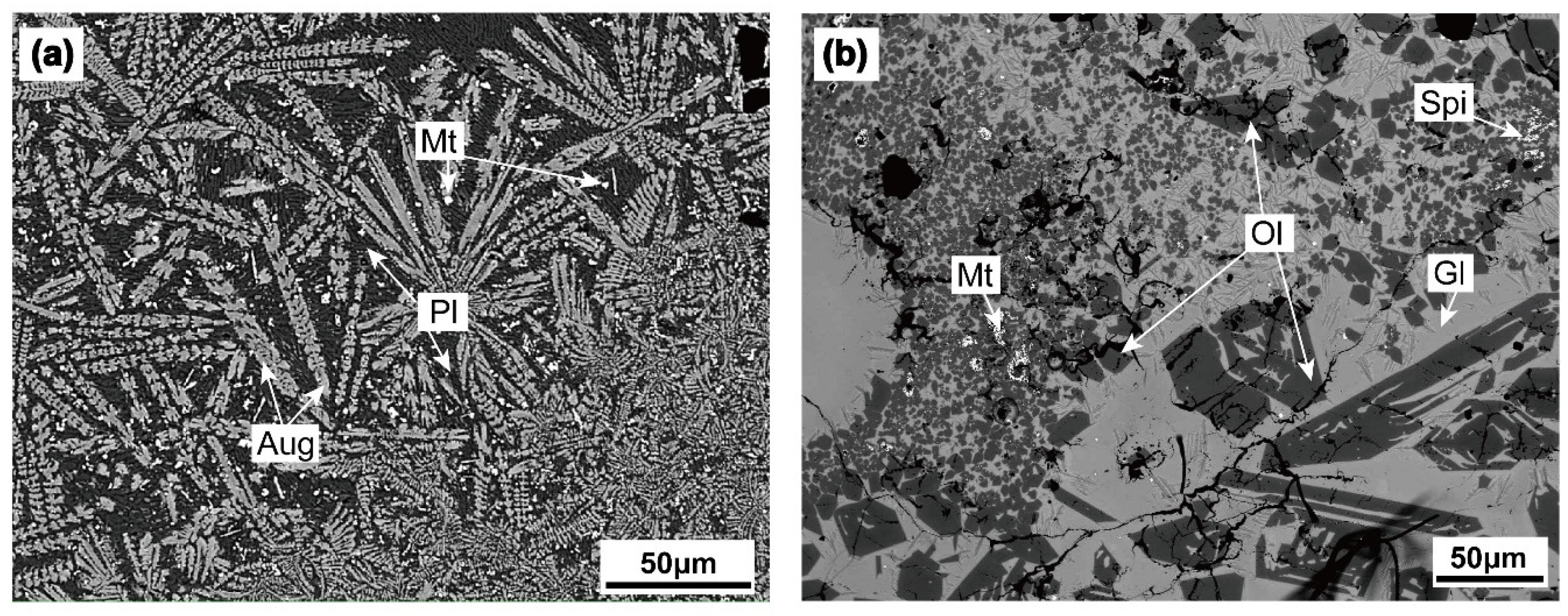The image is a highly magnified, microscopic level diagram composed of two black-and-white photographs positioned side by side. Each photograph features various labels and identifiers pointing to specific areas within the images. The left-side image is labeled "(A)" in the upper right corner, and it includes annotations such as "MT," pointing to a distinct white speckle slightly above the center, and "PL," pointing to two different regions below. The right-side image is labeled "(B)" in the top left corner. Both images include scale indicators in the bottom right corner, denoted as 50 units of an unspecified but presumably very small measurement. Despite the detailed labeling and pointing arrows, the exact subject or nature of the images remains unclear.